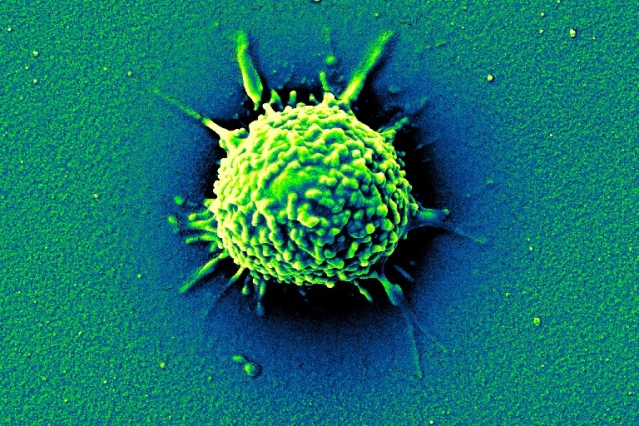This image presents a highly detailed, color-enhanced microscopic view, possibly of a gelatinous, viscous substance or organism, whose exact nature—biological or synthetic—remains ambiguous. Predominantly centered in the composition, this organism or structure is hyper-colored with bright lime green hues accentuating its raised regions, while receded areas shift from mid-blue to an almost black shade. The foreground features a granular surface, speckled and texture-rich, also rendered in various shades of green and spotted with light green specks.

This central structure, round and intricate, bears a resemblance to a virus, characterized by its bumpy, small golden surface and radial protrusions of irregular shapes, sizes, and colors. Additional smaller, light yellow round structures dot the upper and side regions of the image, contributing further to its scientific allure. The image lacks any textual elements or borders, with its artistic style leaning into scientific slide photography, combining elements of photographic realism and high-magnification imaging. The overall aesthetic suggests a deliberate, computer-assisted enhancement to emphasize the striking contrasts and details within this speculative microcosm.